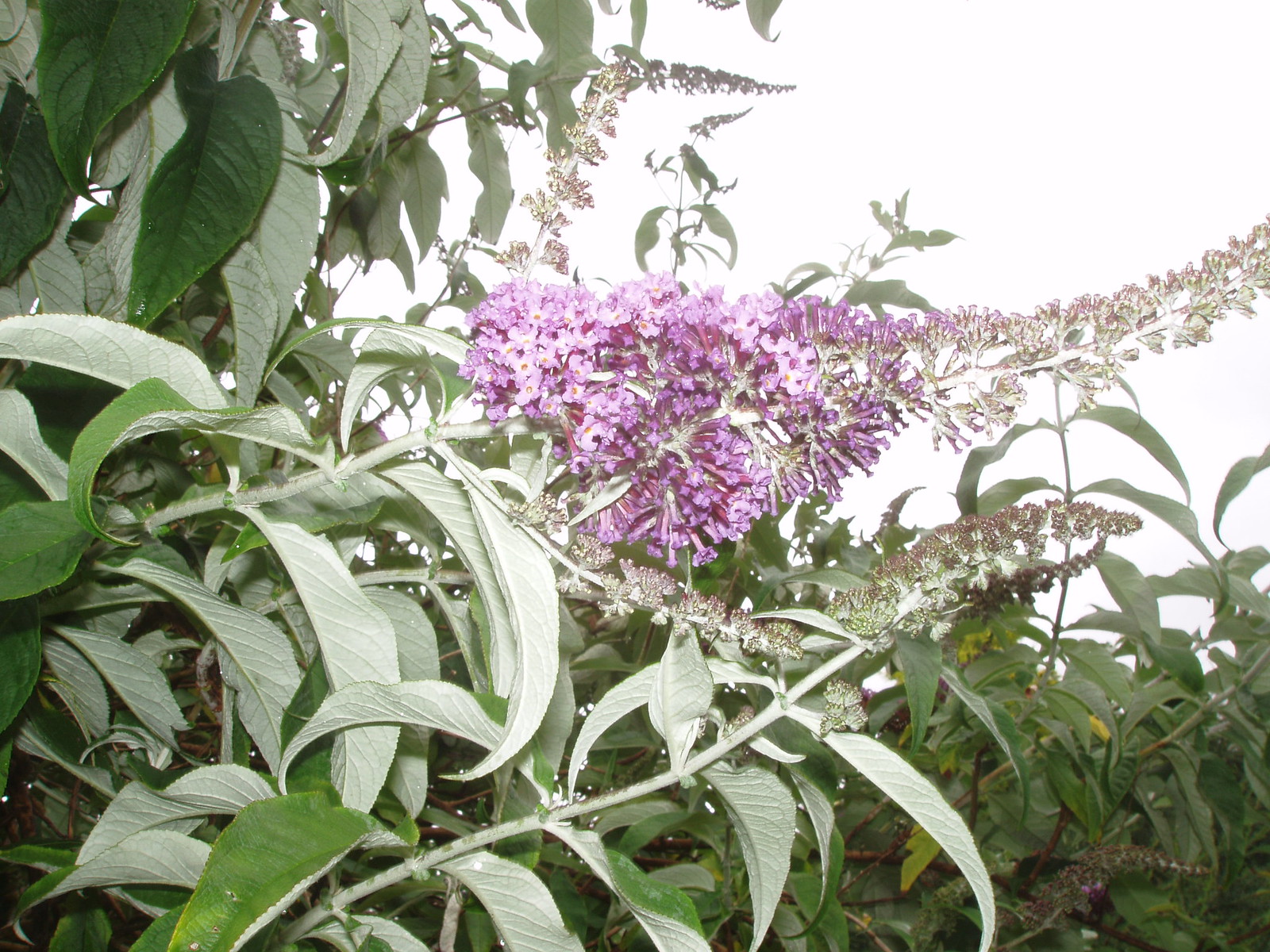The image is a close-up of a flowering plant with distinct, long, and downward-curling leaves. These leaves exhibit a gradient in color, being dark green on the top and light green on the underside. Central to the image is a prominent cluster of lilac blossoms, radiating a range of hues from light purple and pink to fuchsia. The blossoms on the main flower are densely packed and taper off towards the tip where they become lighter and less thick. Surrounding this central flower are several less developed blossoms, either not yet fully blooming or past their peak. In the background, a dense thicket of mature lilac foliage suggests the lateness of the season, with the leaves framing the scene and casting silhouettes against a bright, hazy gray sky. The top left corner features additional clusters of the same plant, echoing the complex interplay of leaves and flowers in the main focus, while the lower right corner shows a more distant view where no flowers are present, highlighting the dark green of the foliage.